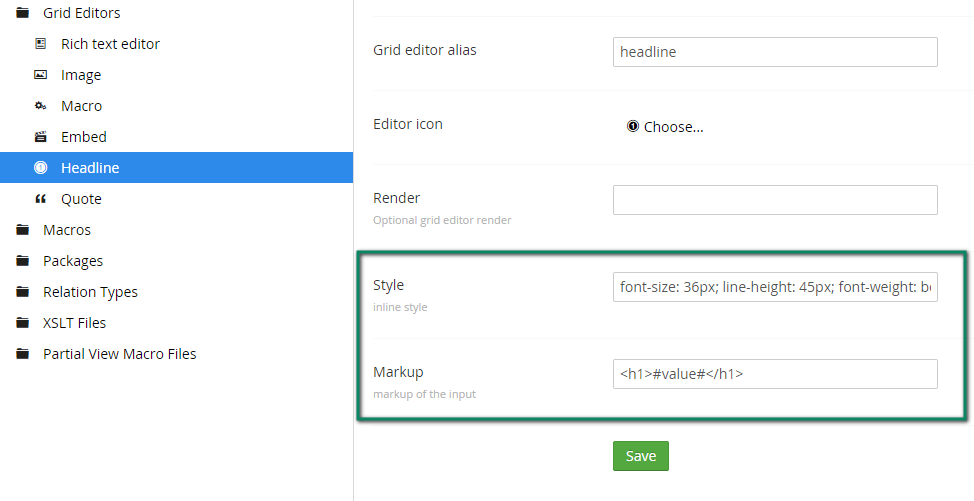Here is a cleaned-up and detailed caption for the image:

---

The image depicts the interface of a grid editor website. On the right side of the screen, a panel displays the details of the item being edited. This panel includes sections for entering a headline, selecting an icon, and a text box adjacent to a render option labeled "Optional Grid Editor Render." Below this, a rectangle with a green border highlights style settings that specify a font size of 36 pixels, a line height of 30 to 45 pixels, and font weight. Further down, there is a text box containing markup with the syntax `[h1]#value#[h1]`. Beneath this markup section, a "Save" button is prominently displayed within a lime-green rectangle.

On the left side of the screen, various settings are available: "Rich Text Editor," "Image," "Macro," "Headline," and "Quote." The "Headline" option is highlighted in blue, indicating that it's currently selected. Additionally, there are folders labeled "Macros," "Packages," "Relation Types," and "XSLT Files," suggesting organizational categories within the editor.

---